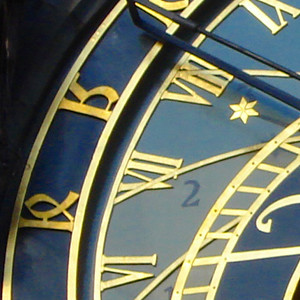This detailed close-up image captures the upper left quadrant of an ornate clock face. Prominently displayed are the Roman numerals VI, VII, VIII, and IX, rendered in a luxurious gold color that contrasts vividly against the rich navy blue background. The clock face is elegantly bordered in black, enhancing its classic appeal. Additionally, intricate yellow designs, including a distinct star symbol, embellish the face, adding a touch of sophistication and artistry to the overall composition.